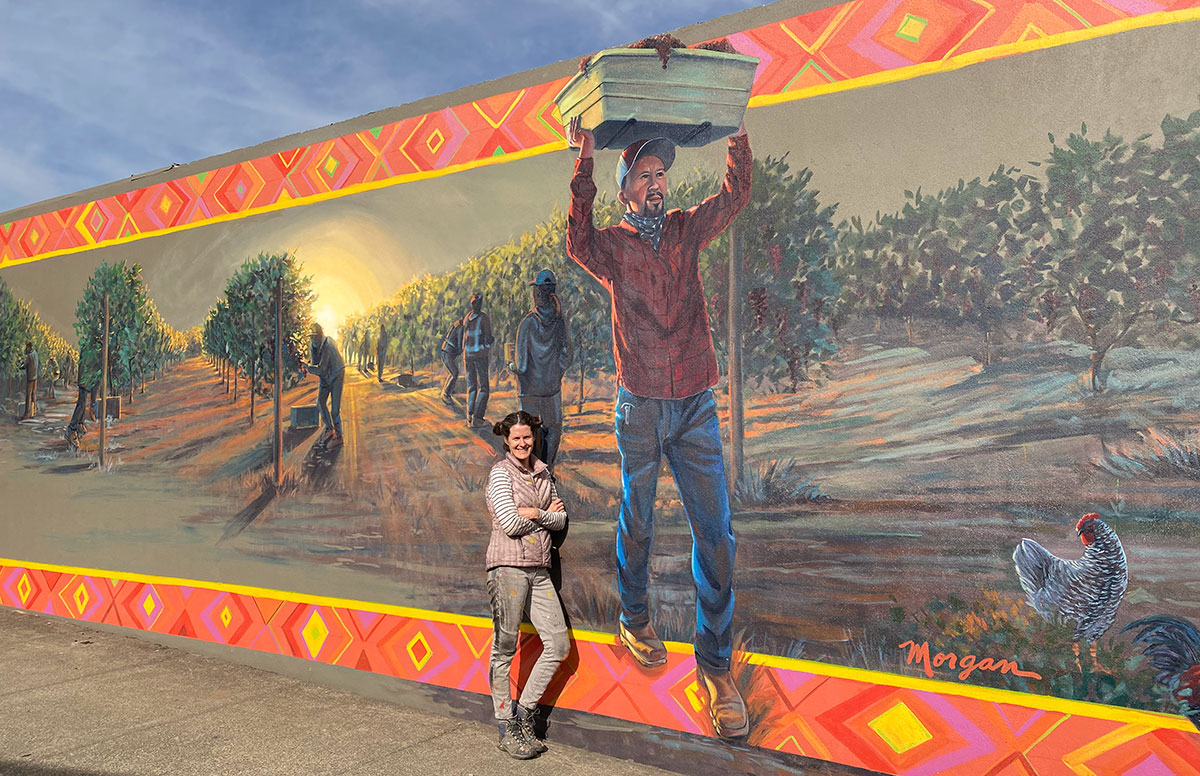The image is a horizontally aligned rectangular picture showcasing a large, tall stone wall adorned with an intricate mural. In the upper left portion of the image, a bright blue sky with feathery white clouds is visible. The mural, framed by a pebbled sidewalk in the lower left corner, is highly detailed and features an agricultural theme.

The mural's upper and lower borders are comprised of yellow and purple diamond patterns set against a coral background. The main section of the mural depicts a vibrant scene of vineyard workers harvesting grapes. Rows of green trees stretch into the background, bathed in the warm light of either a rising or setting sun. The workers, shadowed by the sunlight, are dressed in various colors, including blue, brown, and bright safety vests. Among them, a prominently painted man stands out. He is dressed in blue jeans, a long-sleeve red shirt, work boots, and a bandana around his neck. A large metal tin, filled with plants or flowers, rests on his head. A small rooster stands near him in the lower right corner of the mural, next to the signature 'Morgan'.

In the foreground, an actual woman is leaning against the wall, potentially the artist of the mural. She has her hair styled in two pigtails reminiscent of Princess Leia, wears a brown vest over a striped shirt, gray pants, and work boots. She stands with her arms folded, smiling at the camera, her presence blending seamlessly with the painted scene behind her.